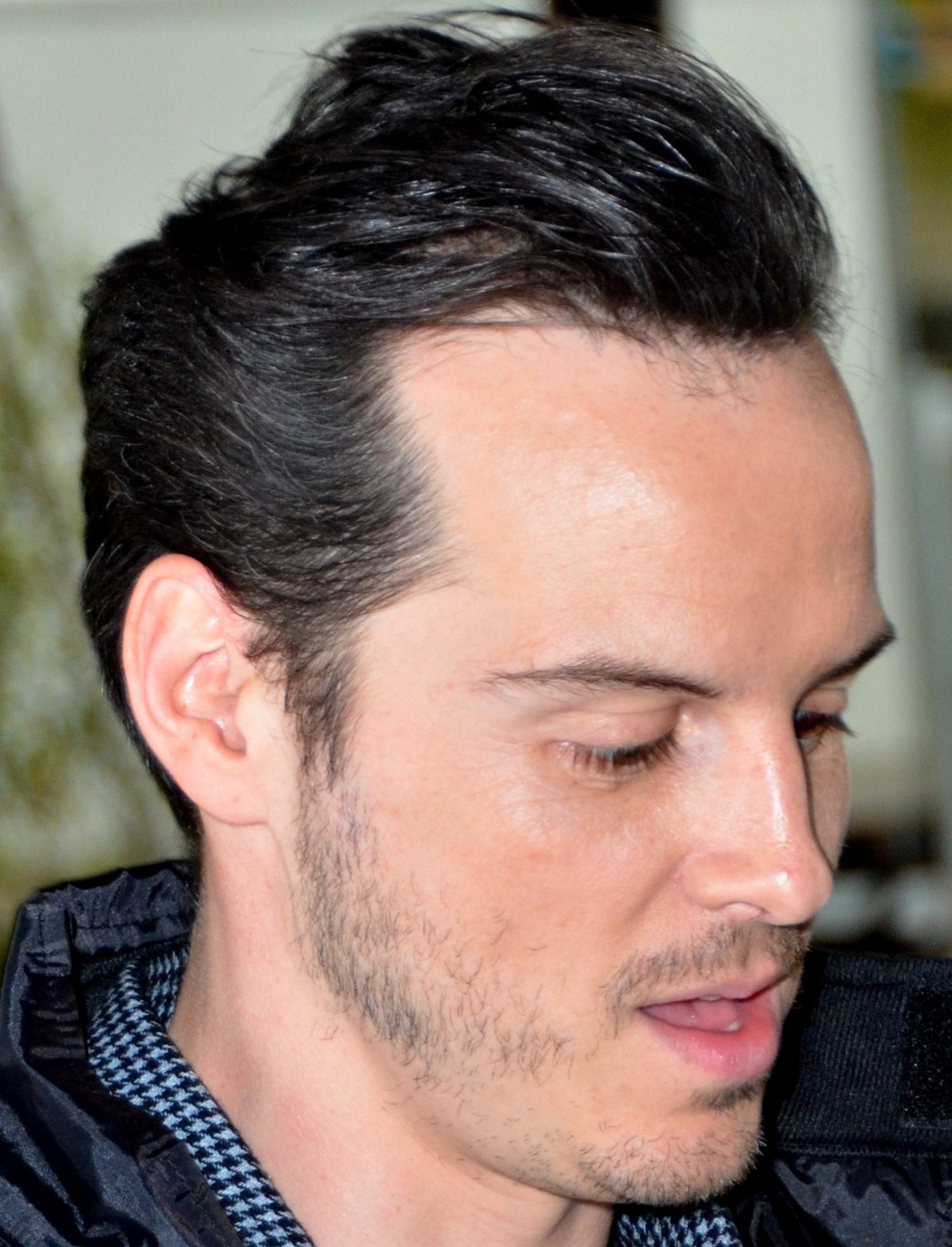A detailed close-up photo reveals a young man, possibly in his early 30s, with dark black hair that is short on the sides and combed straight back, hinting at a pattern baldness. He has scraggly sideburns, a short mustache, and a scruffy beard on his chin and cheekbones. The man's expression appears slightly surprised, with his mouth partially open as he looks down and to his left, his face at a slight angle. He is dressed in a patterned black and white collared shirt underneath a dark, lightweight windbreaker jacket. The background is blurred, offering an indistinct view with off-white and green tones, possibly indicating a room with tan walls.